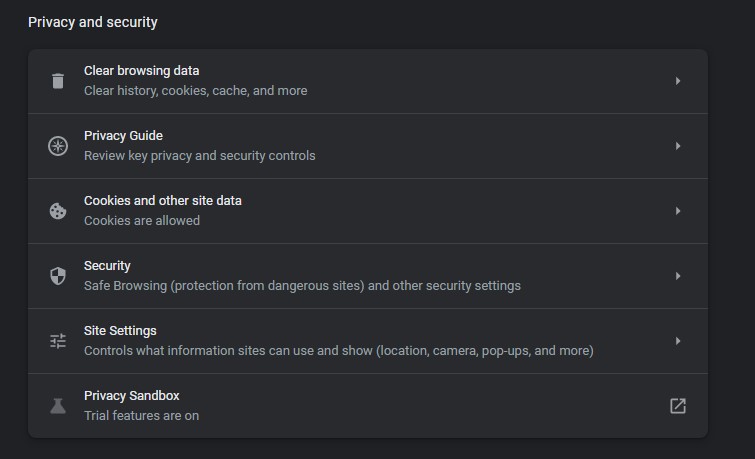The image depicts a screenshot of a "Privacy and Security" settings page with a black background. Centrally positioned within an inner rectangle, the content is divided into six smaller rectangular sections. Each section has a title and a brief descriptive sentence beneath it, accompanied by an icon on the left and a right-facing arrow on the far right.

1. **Clear Browsing Data** - Icon of a trash can; description reads, "Clear history, cookies, cache, and more."
2. **Privacy Guide** - Description reads, "Review key privacy and security controls."
3. **Cookies and Other Site Data** - Description is partially visible but suggests management of cookies and related data.
4. **Security** - Likely includes settings pertaining to securing the user's data.
5. **Site Settings** - Pertains to configuring site-specific privacy and security settings.
6. **Privacy Sandbox** - Features an icon that resembles an upload/download button, with an arrow pointing to the right; likely related to refined privacy features and descriptions underneath. 

Each section is clearly delineated, facilitating easy navigation and understanding of the various privacy and security options available to the user.